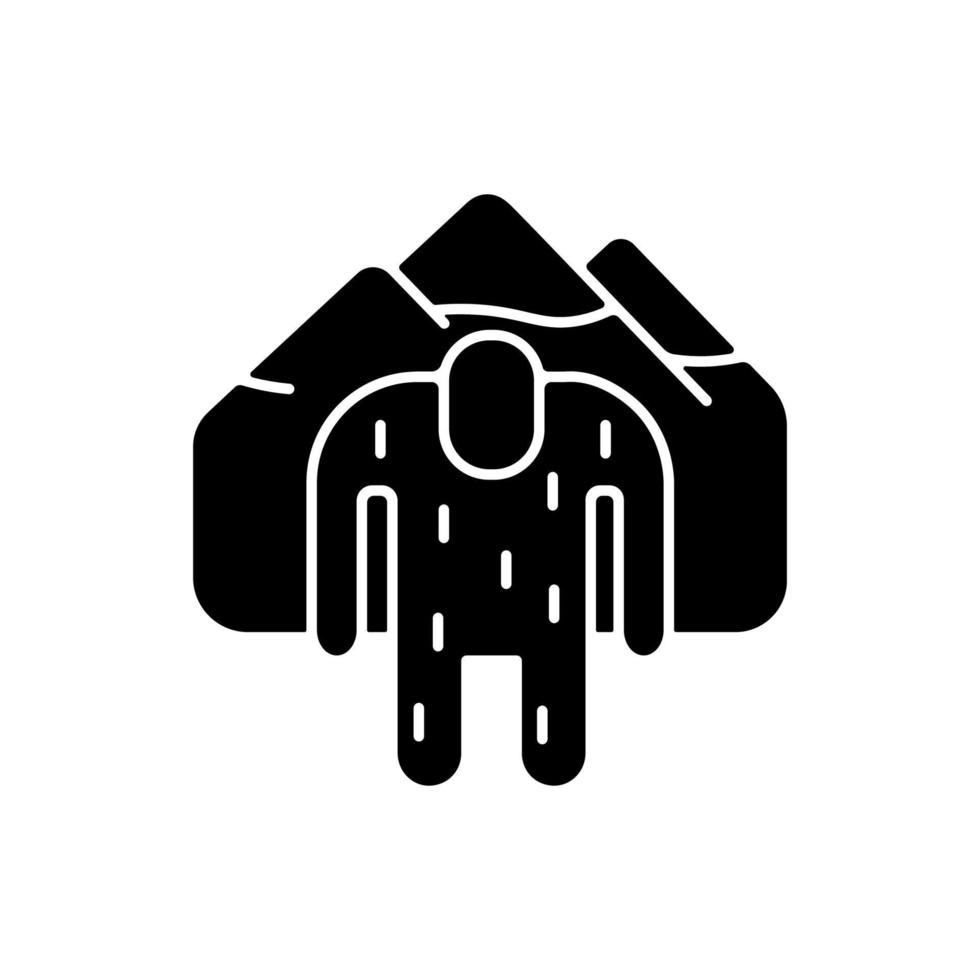This detailed illustration is a digital, black-and-white vector drawing. The image prominently features three mountain peaks in the background, with the central peak being the tallest, flanked by a slightly shorter and a significantly shorter peak. The mountains have contouring lines that suggest their rugged terrain.

In the foreground, there's a human-like figure, depicted with an oval head, two arms, and two legs, identified by a series of short, white vertical stripes across its body and legs, resembling polka-dot lines. The figure seems to be symbolically carrying the mountains on its back, as it is crouched down with arms positioned as though supporting a massive weight. The figure’s lack of facial features and detailed anatomy gives it an abstract, symbolic appearance, reminiscent of a logo. Overall, the illustration conveys a thought-provoking scene of a person bearing the weight of mountains, using simple yet evocative black silhouettes with white highlights.